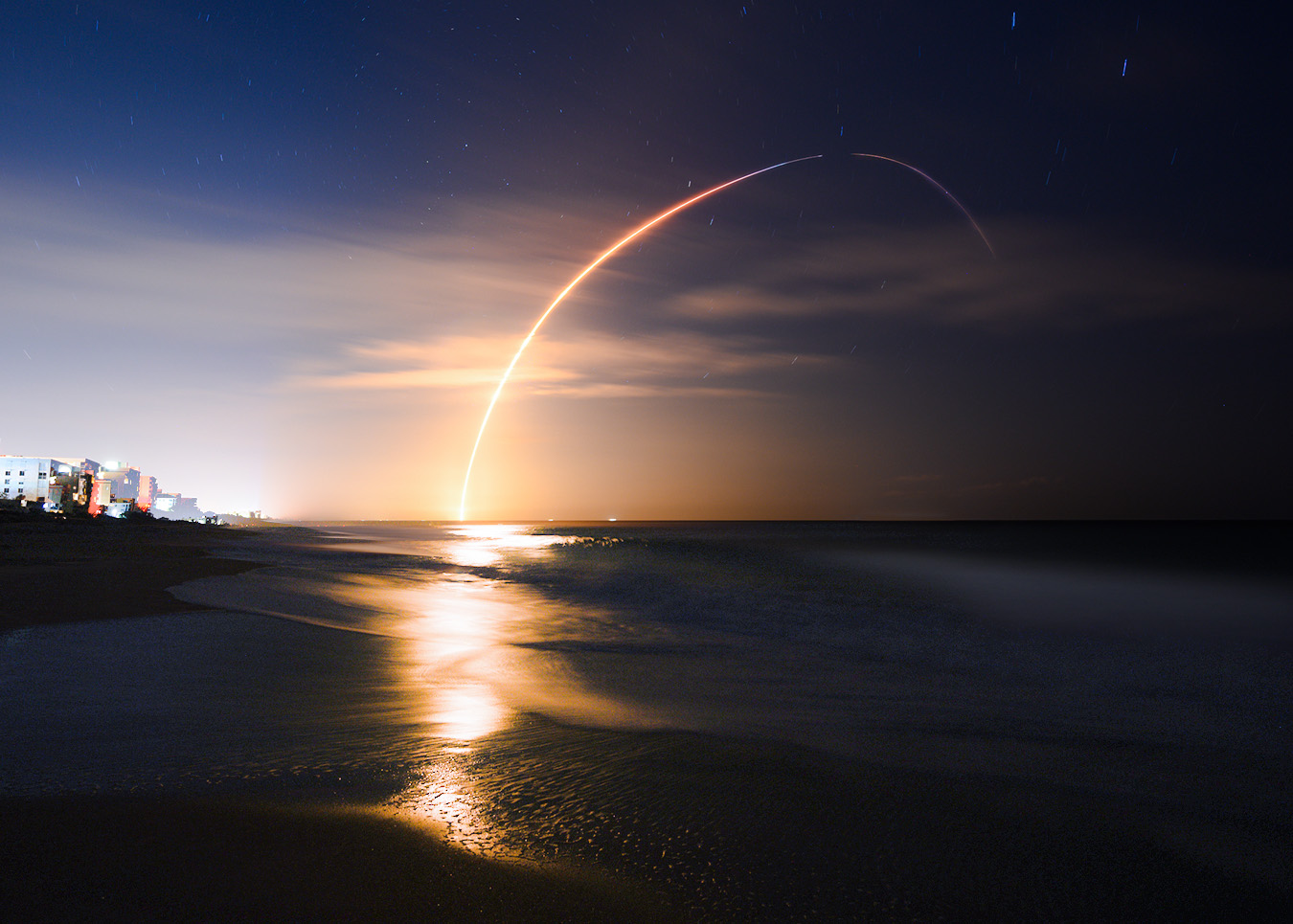In this professional night photograph, a breathtaking beachfront scene unfolds under a twilight sky. The image captures a vivid streak of light, possibly from a lightning strike or a missile launch, piercing through the purplish, orange, and reddish sky, which is dotted with wispy clouds and stars. On the left, a well-lit resort or hotel complex, with its lights glowing in shades of yellow, orange, and red, stands out against the darkening backdrop. The shoreline, with its gently washing waves, is illuminated enough to reveal the wet sand glistening under the fading light. The intricate details of the buildings are faint but discernible, creating a serene yet dramatic coastal ambiance.